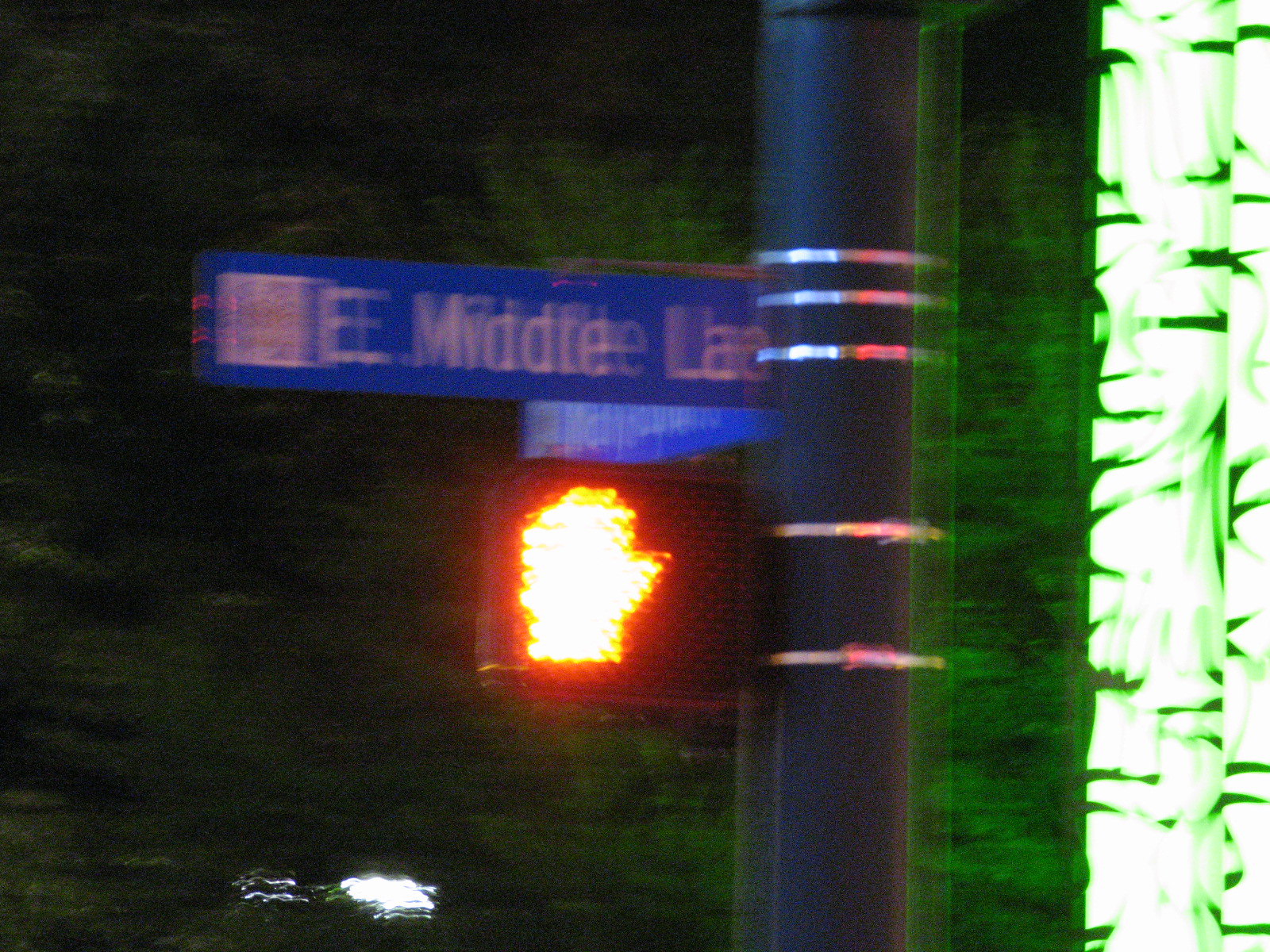This image captures a somewhat blurry, low-quality photograph of a street intersection marked by a crosswalk "Don't Walk" sign and a street name sign. Dominating the right side of the photo is a dark grey to black pole, adorned with several silver metal straps—three at the top and two at the bottom—securing the signage. The street sign, mounted at the upper section of the pole, reads "East Middle LA" on a standard blue background, though parts of the text are obscured and difficult to make out. Adjacent to this, another sign, angled diagonally and unreadable, adds depth to the scene. The "Don't Walk" sign is lit up with an orange hand symbol, clearly indicating a stop. It's presented within a black box where the textured lights are visible. In the blurred background, indistinguishable foliage suggests a nature-rich environment. The overall color palette consists of blues, reds, greens, and a mix of dark grey, black, and silver from the pole and straps.